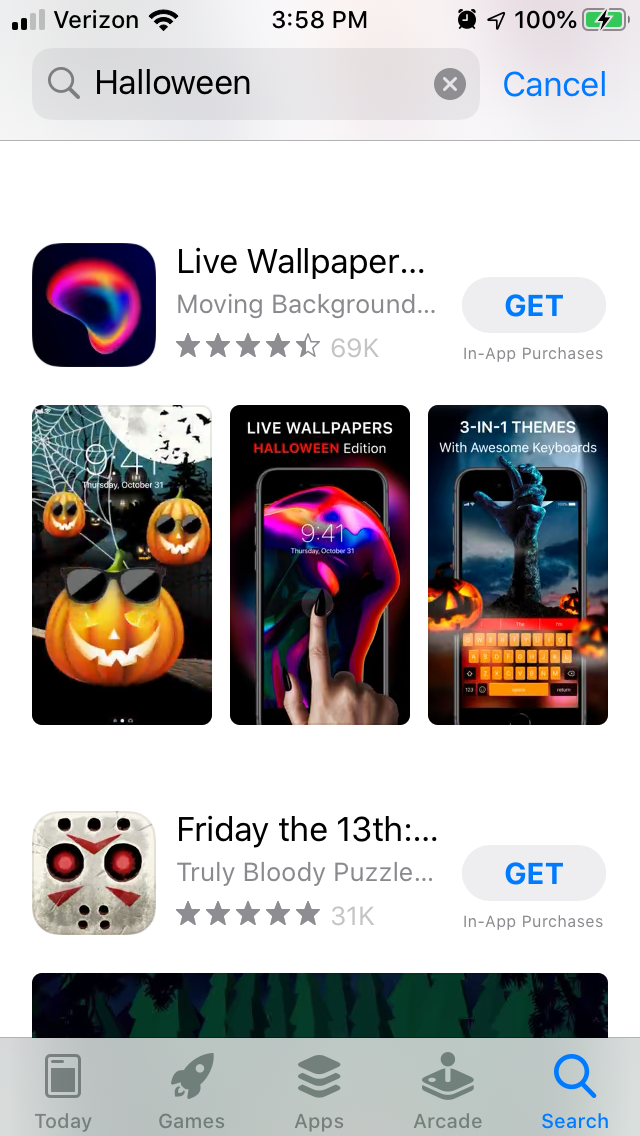This screenshot captures a display of a smartphone screen featuring a selection of live wallpapers and themed apps. At the top left corner, there's a wallpaper icon resembling an orb, which is a blend of orange, red, lavender, and blue colors, indicating its dynamic and movable nature. In the center of the screen, prominently displayed text reads "Live Wallpaper - Moving Background," which boasts a rating of 4.5 stars out of 5, backed by approximately 69,000 reviews. To the right, a “Get” button indicates the availability for download with in-app purchases.

Below this section, the screenshot showcases various wallpaper options. The first one is themed for Halloween. The central wallpaper features the aforementioned dynamic orb with an additional tag indicating it's a "Halloween Edition." The third wallpaper is also Halloween-themed, promoting "3-in-1 themes with awesome keyboards," all featuring classic Halloween imagery like pumpkins and orange hues.

Further down, there's a featured app section highlighting "Friday the 13th," adorned with the iconic mask of the main character from the franchise. This app is marketed as a "Truly Bloody Puzzle," earning a perfect rating of 5 out of 5 stars from 31,000 votes, and it also comes with a "Get" button, suggesting in-app purchases.

At the bottom of the screen, a navigation bar displays tabs for "Today," "Games," "Apps," "Arcade," and "Search," with the search function currently highlighted.